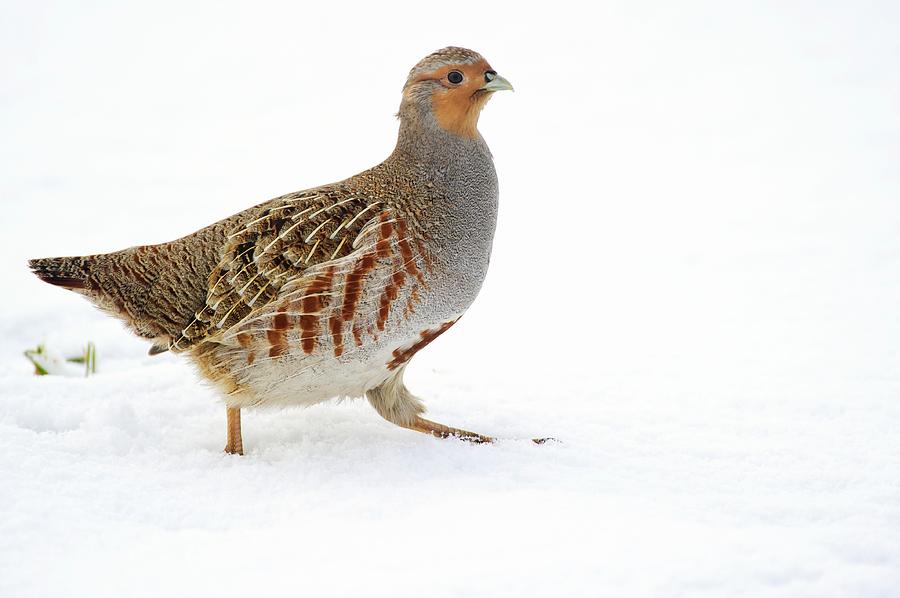In this detailed image, we see a bird from the pheasant family walking across a snowy field, where the background is predominantly white, with a few blades of grass poking through the snow. The bird is centrally positioned, facing right with its left foot slightly lifted and its right foot firmly planted on the ground. 

The bird's head is primarily gray with a tint of brown around the eyes, leading up to a small broad gray beak with a black tip. The eyes are dark brown, almost black. The top of its head and its neck are gray, transitioning to a combination of tan and brown near its face and neck area. The chest feathers display a mix of black and white, creating a speckled, almost grayish pattern, while the belly feathers are white. 

Its wings are a striking feature, with a base color ranging from dark brown to black, interspersed with rust-colored and white stripes. The upper parts of the wings are darker while the lower parts exhibit lighter brown and white feathering. The tail of the bird is short, displaying a mix of darker and lighter feathers, primarily brown with hints of black and tan.

The legs and feet of the bird are light orange, blending into the surrounding snow. The overall impression is of a bird with dense, thick feathering, adapted for its cold environment.